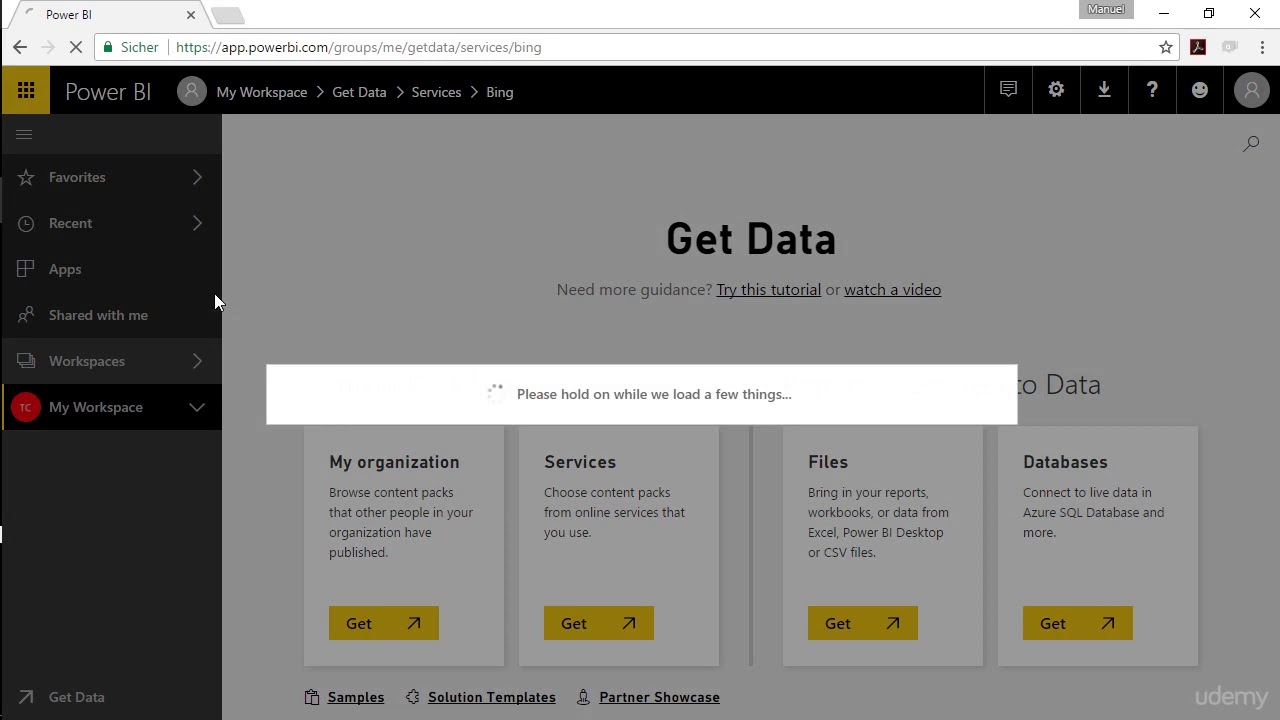This screenshot from a computer screen captures a Power BI webpage. At the top of the screen, the URL displayed is "https://app.powerbi.com/groups/me/getdata/service/Bing". The top section features a black header area with a yellow box that contains a black cube composed of smaller squares. Next to it, the text "Power BI" appears in white, followed by a human icon and several navigation options: "My workspace," "Get Data," "Services," and "Bing."

In the central section of the webpage, there is prominent black text displaying "Get Data." Below this, an advisory message reads, "Need more guidance? Try this tutorial or watch a video." A loading prompt asks users to "Please hold on while we load a few things..." within a white rectangle, accompanied by a spinning circle indicator.